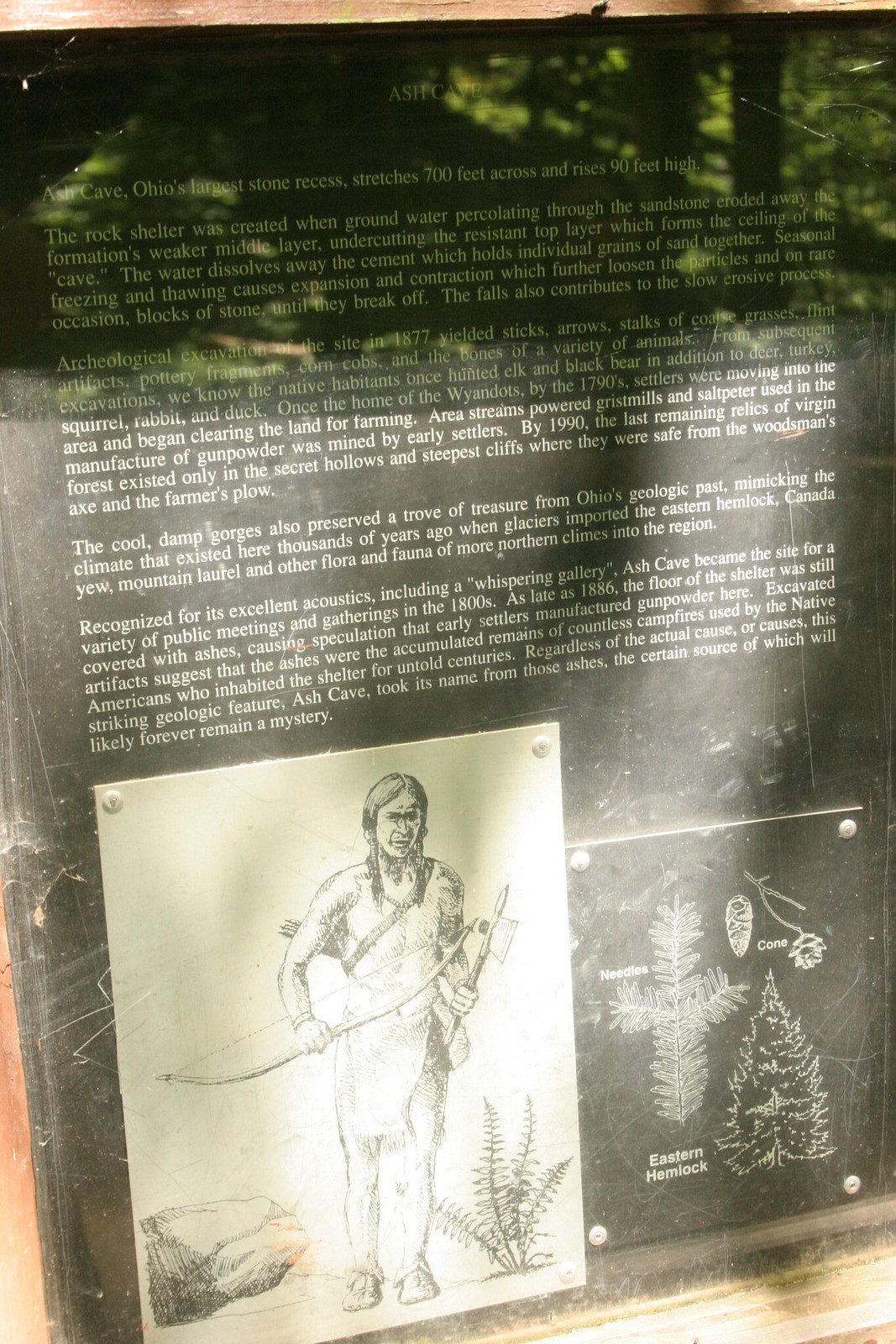This tall, rectangular image features an informative sign at a museum, angled such that the left side appears closer than the right, and slightly tilted to the left. Dominating most of the image, the sign is topped with the bold, all-capitalized title "ASH CAVE." Below this heading, five paragraphs of white text describe the area's geological and historical significance. The text explains that Ash Cave, Ohio's largest stone recess, stretches 700 feet across and rises 90 feet high. It discusses the natural erosive processes involving groundwater, seasonal freezing and thawing, and rock falls that have shaped the cave.

At the bottom left corner of the sign, there's a bolted-on black-and-white drawing of a Native American man. He is minimally clothed, holding a bow and arrow in one hand and a hatchet in the other, with additional arrows visible behind his back. The figure stands with a plant featuring several spikes at his feet, and further to the right of him are diagrams showcasing various kinds of leaves and plants. The background of the sign also includes a wooded area filled with green trees, creating a naturalistic setting for the detailed and informative display.